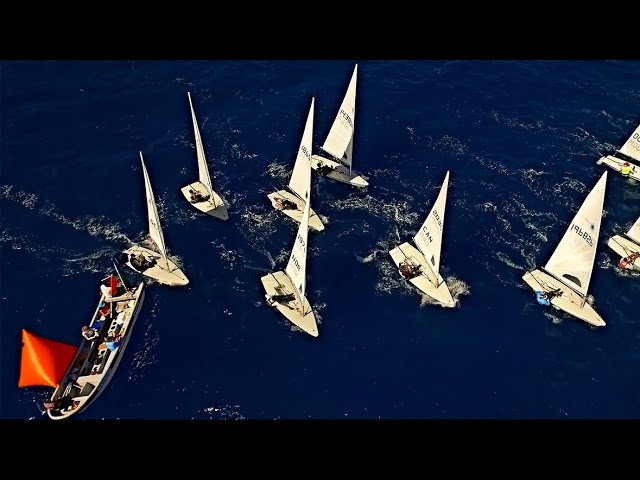This is an aerial photograph of an outdoor scene illustrating a sailing race, or regatta, viewed horizontally. The dark navy blue ocean fills the center of the image, flanked by black bars at the top and bottom. The ocean appears lively with sailing activity, as white waves and trails highlight the movement of the vessels. Central to the scene are about seven to nine small sailboats, each featuring pristine white sails marked with large numbers, like '196826'. The boats, streamlined and triangular in shape, have a creamy body and are sailing towards the bottom right corner of the photograph. Positioned near the lower left, there’s a longer, flatter boat, possibly a record-keeping vessel, accompanied by an inflated orange buoy. This boat carries some people, visible along with supplies and equipment, hinting at its role in the event. The image captures the dynamic essence of the race, with sailors actively maneuvering their boats amid a good wind.